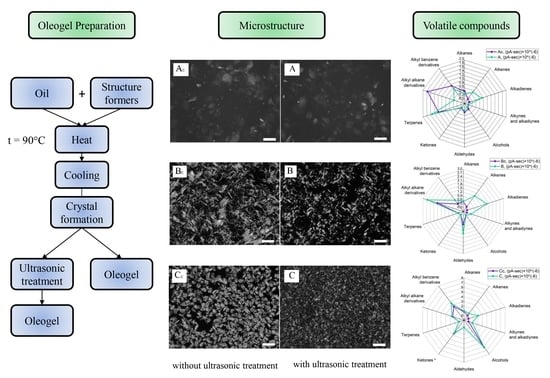The diagram is organized into three vertically aligned sections, each with a green title box containing the key terms: "Oleogel Preparation," "Microstructure," and "Volatile Compounds."

In the first section, titled "Oleogel Preparation," it begins with a visual flowchart. The process starts with two blue text boxes labeled "oil" and "structure formers," connected by a plus sign. An arrow leads down to three steps: "heat," "cooling," and "crystal formation." Further down, crystal formation branches into "ultrasonic treatment" and "oleogel," both converting into oleogel eventually.

The second section, titled "Microstructure," features a comparative analysis of microscopic images. There are three sets of side-by-side images labeled A, B, and C, each pair showing untreated samples on the left and ultrasonically treated samples on the right. The images are primarily black with varying concentrations of a white, cloud-like structure. In general, the treated samples display a denser white structure compared to their untreated counterparts. Descriptive text clarifies that the left three images are without ultrasonic treatment, while the right three are with ultrasonic treatment.

The third section, titled "Volatile Compounds," displays three spiderweb-like diagrams, each with interconnected lines in light blue and purple arranged in different patterns. These diagrams are surrounded by descriptive text detailing the various elements and compounds analyzed.

Overall, the diagram comprehensively details the preparation process, microstructural differences due to ultrasonic treatment, and the composition of volatile compounds, offering a detailed and visually structured presentation suitable for a scientific context.